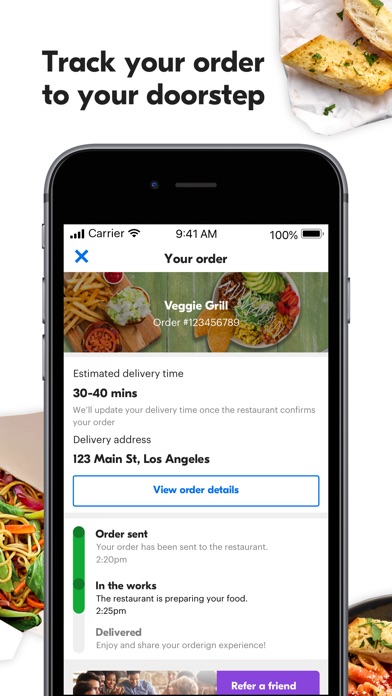This is an image of a website interface designed for tracking food orders. The background is predominantly white with black text. Approximately an inch below the top edge of the image, and aligned to the left, the text "Track Your Order" is prominently displayed in bold black lettering. Directly beneath it, in a smaller font, is the phrase "to your doorstep."

In the top right corner of the image, there appears to be a graphical depiction of a burger. Partially visible, a burger wrapper extends about two inches left from the corner and slightly downward. Above and to the right, there are two pieces of bread angled downward with a small garnish of green herbs on top. Additionally, the bottom right corner shows a portion of a round serving tray, roughly an inch in diameter, holding another piece of bread along with an arrangement of orange noodles, of which three are visible.

Towards the bottom left of the image, about an inch from the base and extending upward for another two inches, there is a small section of a salad arranged horizontally from left to right. 

Centrally positioned underneath the "to your doorstep" text, there is an outline resembling a smartphone. The top portion of the phone, which is white-bordered, displays the common indicators such as the carrier name, current time in the center, and battery status on the right side. Beneath the time display, the text "Your Order" is visible in black, along with a photograph featuring a variety of food items. On the left side of the image, the foods shown include fries, a hamburger with a tomato slice, and some salad. The right side displays items such as tacos and assorted vegetables, with "Veggie Grill" labeled across it.

Finally, within the smartphone interface, the detailed order information is presented, including estimated delivery time, the delivery address, and order specifics. At the bottom of this interface, there is a button labeled "Track Order."